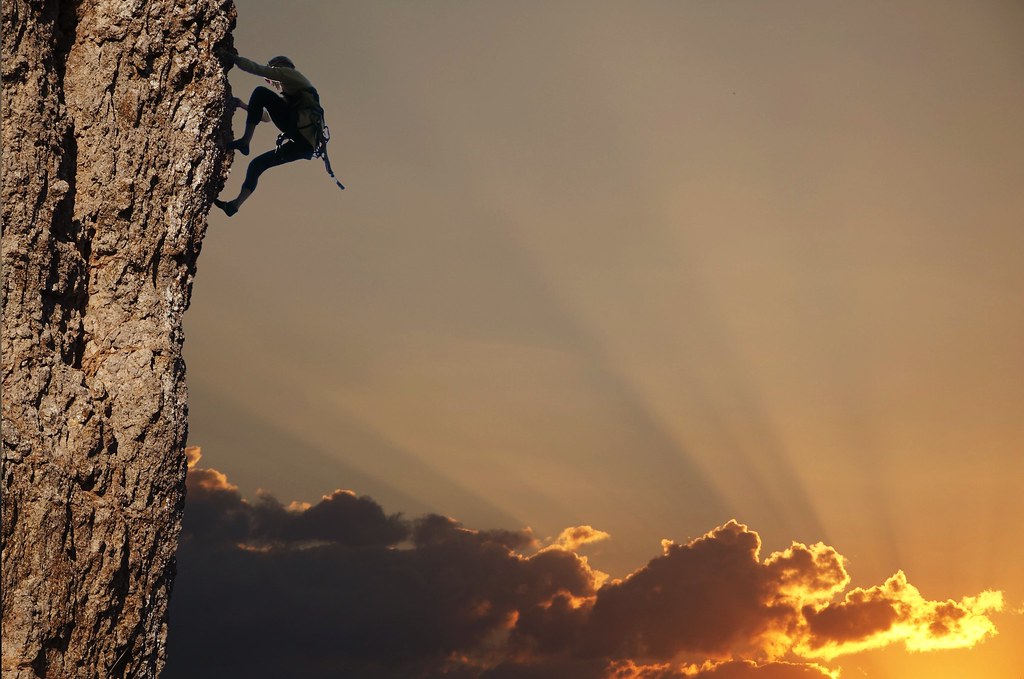The photograph captures a dramatic moment of a man climbing a steep, rough, brown cliff that dominates the left side of the image. The rock face, vertical and slightly angled to the right, presents a challenging ascent. The climber, positioned near the top of the frame, is dressed in a tight black bodysuit and climbing shoes, with equipment strapped around his waist and a stick-shaped object secured to his back. His legs are bent, with one higher than the other, and he grips the rock face with both hands, his face obscured by his arm. The background features a gray sky tinged with the evening's dramatic hues. Black and yellow clouds fill the lower part of the sky, illuminated by bright yellow light rays originating from the bottom right, casting an ethereal glow across the scene.